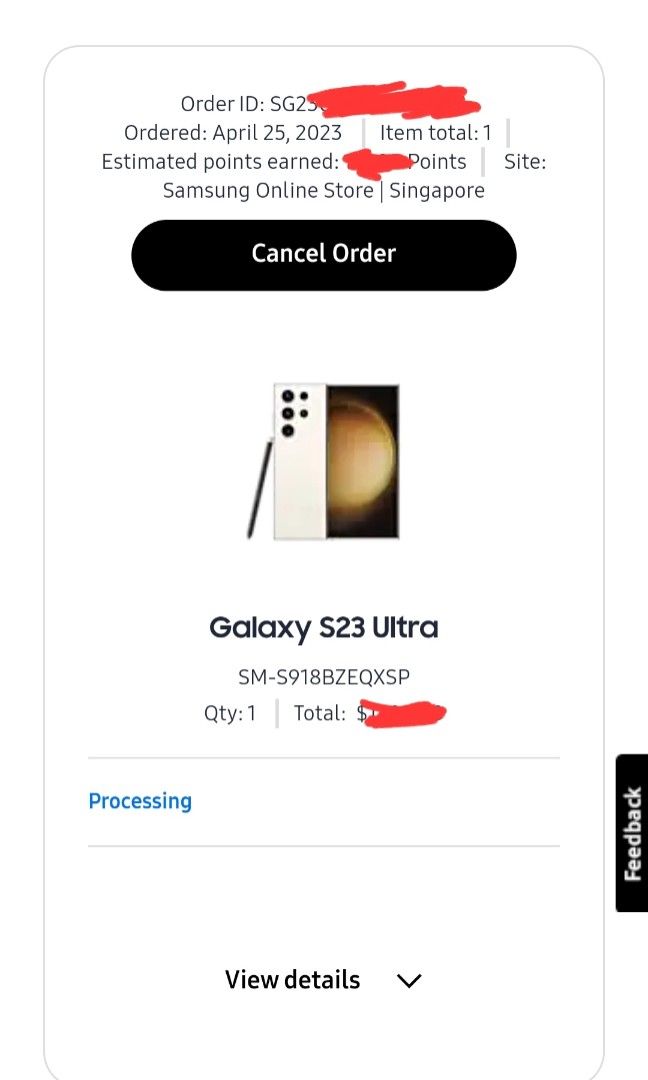The image features a vertically oriented screenshot against a white background, displaying details of an order from the Samsung online store in Singapore. 

At the top of the image, the text reads "Order ID 5g," followed by red scribbles obscuring part of the Order ID for privacy. Below this, the screenshot indicates the order was placed on April 25th, 2023, with an item total of one. The section stating "Estimated points earned" also has parts scribbled out except for the word "points." Adjacent to this, it says "Site: Samsung online store Singapore."

Beneath this information, there is a prominent black button with white text that says "Cancel Order." Below the button, a clear image of the Samsung Galaxy S23 Ultra is displayed, showcasing the smartphone with a stylus pen leaning against it.

The product is identified underneath the image with the text "Galaxy S23 Ultra" followed by the model number "SM-S918BZeqX." Further details indicate the quantity ordered as "1" and the total cost, which has been scribbled out. 

In the section below the product description, the order status is shown in blue text as "Processing." At the center bottom of the image, there's black text stating “View details” accompanied by a downward-pointing arrow. Finally, on the far-right side of the image, another black button with white text reads "Feedback."